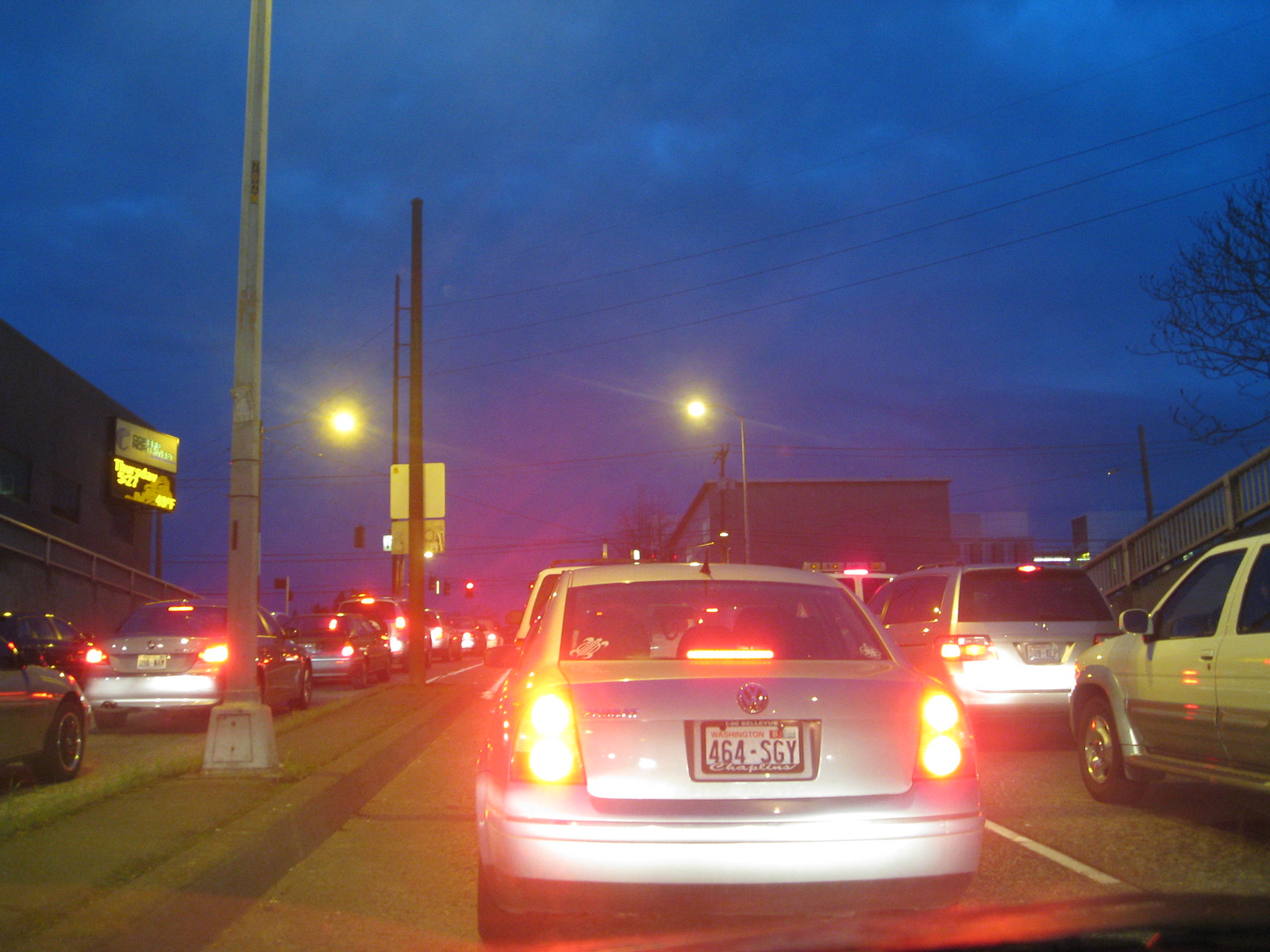This is a detailed nighttime photograph taken from inside a car, looking out through the windshield at a traffic jam. The scene is illuminated by the reddish glow of numerous taillights from the closely packed cars, mostly sedans, suggesting that the vehicles are either stationary or moving slowly. The license plate of the car directly ahead is "464SGY." Above the street, power cables stretch across the road from pole to pole, and several streetlights cast a dim light on the scene. The sky is a dark blue, filled with post-sunset clouds. To the left, there is a blurred yellow sign on a flat-roof building, while on the right, sparse trees with few leaves can be seen. Railings line either side of the road, making it appear as though this section of the street has just emerged from a tunnel.